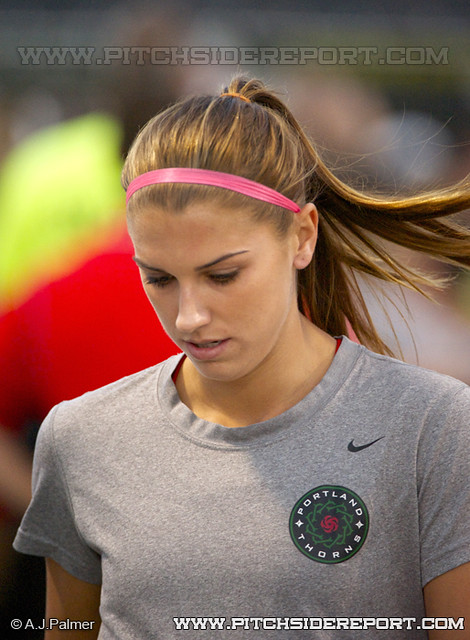This image captures a young female athlete, visibly portrayed from her chest upwards against a blurred background, indicating a public setting with several indistinct figures in the distance. She appears to be in her late teens or early twenties, with her light brown hair pulled back by a noticeable pink headband. She’s looking down, giving a sense of contemplation or focus.

She is clad in a gray short sleeve t-shirt adorned with a circular logo bordered in green, displaying the white text "Portland Thorns." Accompanying this logo is a small black check mark above. Watermarks are prominently visible within the image: "www.pitchsidereport.com" appears transparently along the top and in white text in the bottom right corner, with a copyright notice “A.J. Palmer” displayed in the bottom left. The overall presentation suggests a professional sports context, possibly linked to softball or soccer, given the team's logo and the associated watermarks.